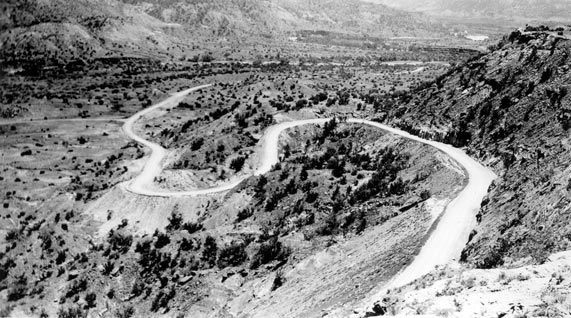This black and white photograph captures a serene desert landscape along a winding hillside road. The image prominently features a steep hill that starts from the bottom right corner and extends all the way to the top right corner. In the far left background, a range of rugged mountains adds depth and contrast to the scene. The valley below is dotted with numerous small shrubs, providing texture to the otherwise barren terrain. The road, appearing as a single lane, begins in the right section of the photograph and meanders gracefully toward the center before curling back and disappearing out of sight toward the middle left. The sky overhead is adorned with scattered clouds, adding a touch of dynamism to this tranquil desert vista.